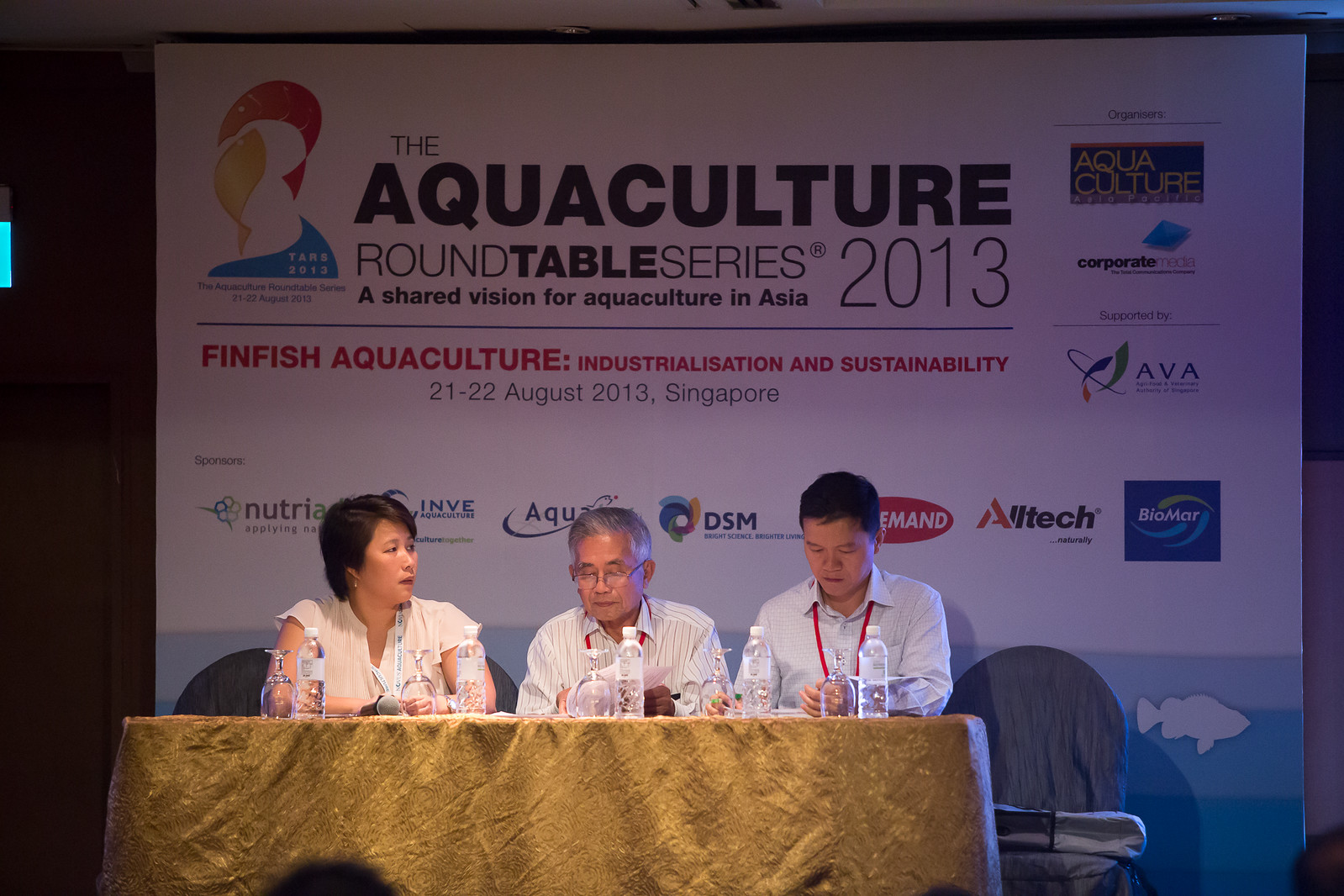The photograph captures a moment at the Aquaculture Roundtable Series 2013 event held on the 21st and 22nd of August 2013 in Singapore. Three individuals, all dressed in white, are seated at a table adorned with a golden tablecloth. The participants include a woman on the left, an older man wearing glasses in the center, and a middle-aged man on the right. Behind them, a large white poster dominates the background, displaying the event's title: "The Aquaculture Roundtable Series 2013: A Shared Vision for Aquaculture in Asia." Additional text on the poster reads, "FinFish Aquaculture Industrialization and Sustainability" alongside the event's dates and location. Below this information, various logos of corporate sponsors are visible, such as Ava, Altech, Biomar, DSM, and others, signifying significant industry support. The table they are seated at holds several water bottles and glasses, indicating they might be in the midst of an intense discussion. The overall scene is bathed in muted lighting with a blue tint possibly emanating from the screen or background design, enhancing the formal yet focused atmosphere of the roundtable.